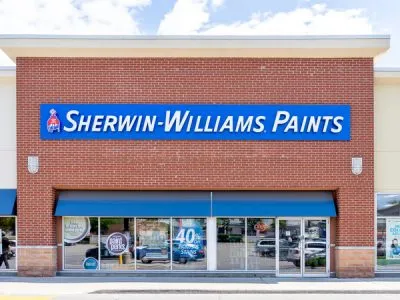In this image, the background features a sky with scattered white clouds. Dominating the foreground is a building with a distinctive two-tone appearance: the top portion is painted white while the lower part is composed of traditional red brick. Prominently displayed on the building is a large blue rectangle featuring a graphic of paint spilling over a globe, accompanied by the words "Sherwin-Williams Paints." Below this sign, there's a blue awning sheltering a series of windows that are difficult to discern due to their small size, possibly containing items or inscriptions behind the glass. 

To the sides of the main building, additional white structures are visible, with the right-hand side displaying more windows or pictures. Within the brick section of the building, there are two pale rectangles, one on each side. The left rectangle seems to include an image of a person, topped with another blue rectangle. Extending towards the street is a light blue-gray pathway, bordered by a white section beneath it and marked by a continuous gray line running from the center-left to the right, paralleled by a yellow line on the far left side.